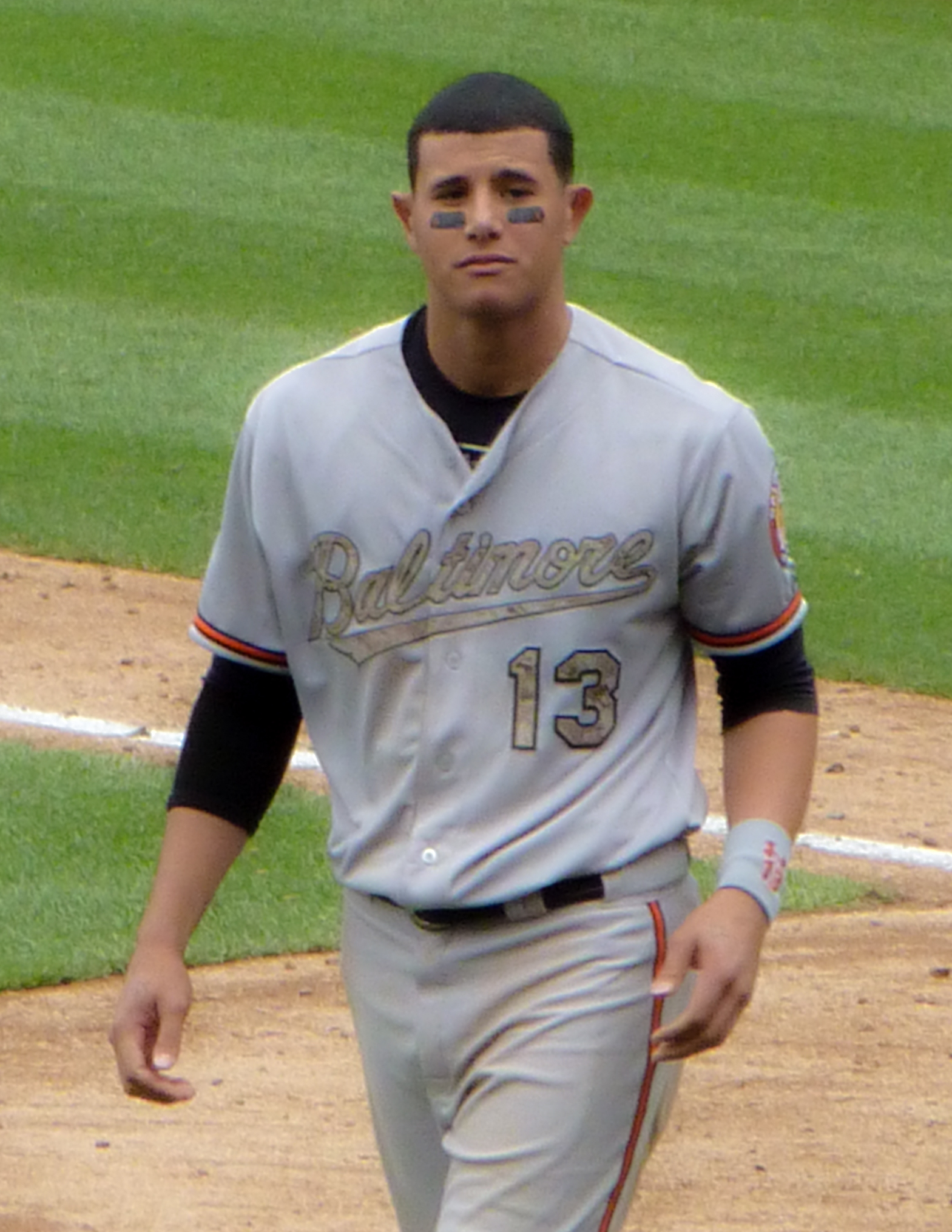The image captures a baseball player from the Baltimore team, identified by the gray jersey with "Baltimore" emblazoned across the chest and the number 13 on its left side. The player sports dark, close-cropped hair and has black eye black under each eye. His uniform includes gray pants with an orange stripe running down the sides and two orange stripes on the short sleeves of the jersey. Underneath his jersey, he wears a tight black long-sleeve undershirt. The player also has a black belt. He is depicted walking across a meticulously maintained baseball field, featuring vivid green grass striped in a pattern of alternating light and dark green, and a diamond composed of brown dirt with white lines. The scene is an outdoor setting, showcasing both the lush field and segment of the baseball diamond.